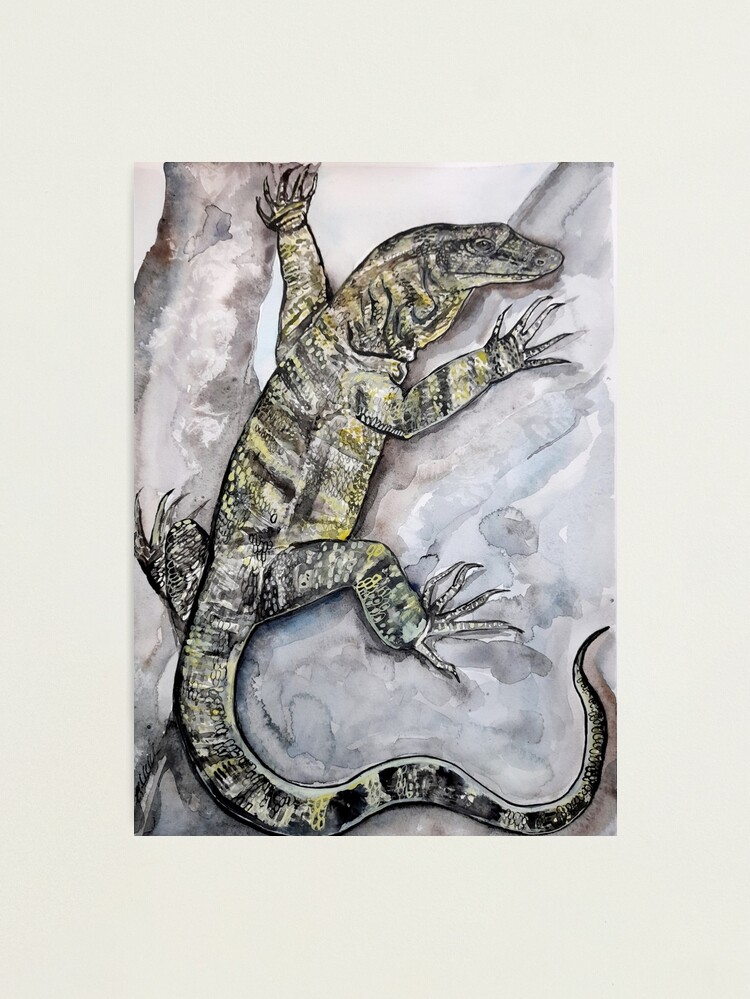The image showcases a detailed watercolor and black-and-white ink illustration of a large lizard, likely an iguana or Komodo dragon. The lizard, which dominates the center of the painting, exhibits a mix of faint black, yellow, gray, green, and gold hues across its scaly hide. Notable features include five long claws on each of its four splayed legs, its right eye visible as it gazes outward, and a closed mouth. Its tail, curving gracefully to the right and bottom, adds a dynamic flow to the composition. The lizard's head is tapered at the nose, with wrinkled neck details, and displays a color gradient from light gray at the top to pale green and white underneath. Accentuating the lizard's form are black stripes and yellow dots along its back and belly. The background, rendered in watercolor, consists of varying tones of brown, ranging from light taupe to dark shades, representing tree branches on which the lizard is perched. Its left legs rest on one branch while the body and right legs extend onto a larger branch, adding depth and natural context to the scene.